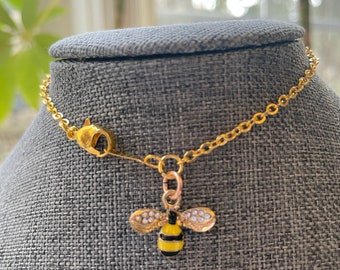The photograph showcases an elegant gold chain necklace displayed on a mannequin. The mannequin, which appears to be made of a light blue to grayish cotton fabric, is headless and only displays the neck area down to the neckline. The focal point of the image is the necklace, which features a pendant of a bee. The bee pendant dangles gracefully from a rose gold chain that is attached to the main gold chain. The bee itself is intricately designed with its wings encrusted with white jewels, and its body displaying two yellow and two black stripes, with a small black head. The background of the image reveals a hint of greenery and a window, suggesting it could be either an outdoor setting or by a window with a view of outdoor scenery. The lighting is bright, further highlighting the exquisite details of the necklace.